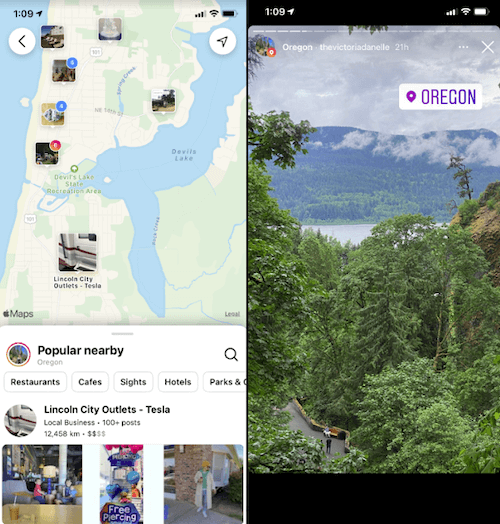This image captures a map highlighting the area of Devil’s Lake and the Devil’s Lake State Recreational Area, suggesting a location in Oregon. The map prominently displays regions of water, indicative of the lake's expansive size, and is bordered by ocean to the west, consistent with the coastal geography of Oregon. Adjacent to the map is an inset image featuring the word "Oregon" in purple lettering. This inset shows a picturesque scene with rolling hills covered in trees, low-lying clouds, and a large body of water, reinforcing the Oregon setting. At the bottom left of the map, there is a "Popular Nearby" section listing local amenities such as restaurants, cafes, sites, hotels, parks, and a notable mention of the Lincoln City Outlets-Tesla.